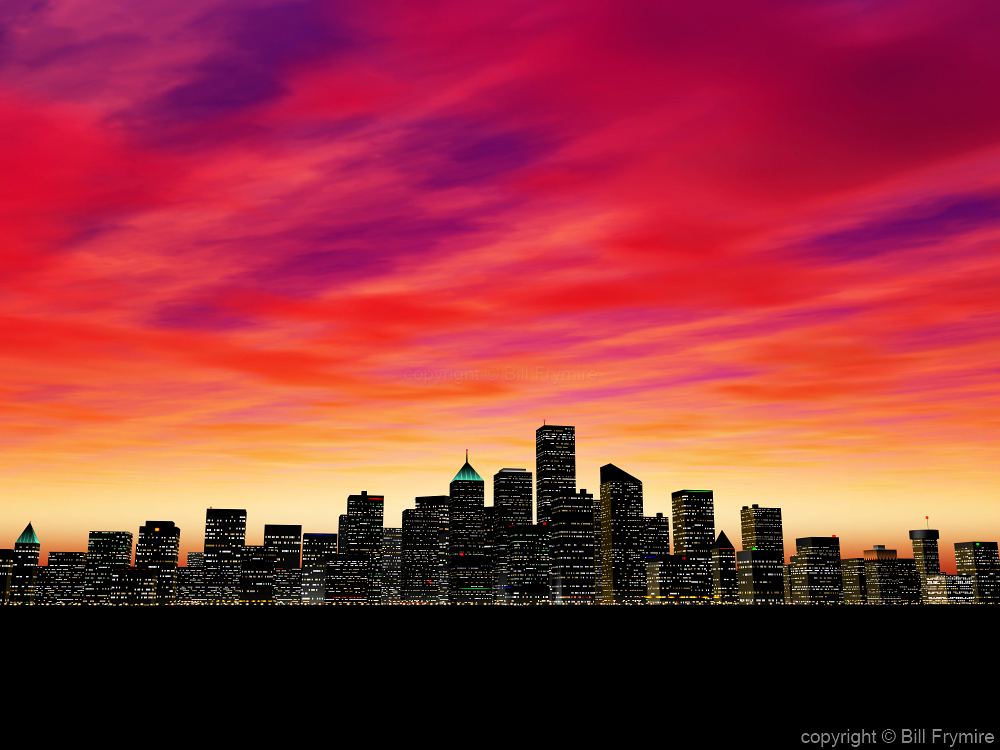This painting portrays a vibrant city skyline under a dramatic sky, potentially capturing either a sunrise or sunset. The upper half of the image features a sky awash with a palette of vivid colors, ranging from deep red and purple to orange, light yellow, and hints of pink and blue, creating a gradient that flows diagnolly from the top right to the bottom left. Beneath this colorful sky is the silhouette of a bustling city, depicted with numerous tall buildings in black. Each building is dotted with white windows, suggesting that the lights are on, indicating either early morning or evening. Among these structures, one building stands out with a triangular top illuminated by green lights, and another is distinguished by an antenna on its roof. The lower third of the painting is a solid black area, possibly representing a waterfront, adding depth to the scene. In the bottom right corner in white text, the copyright notice reads "copyright Bill Freymire."